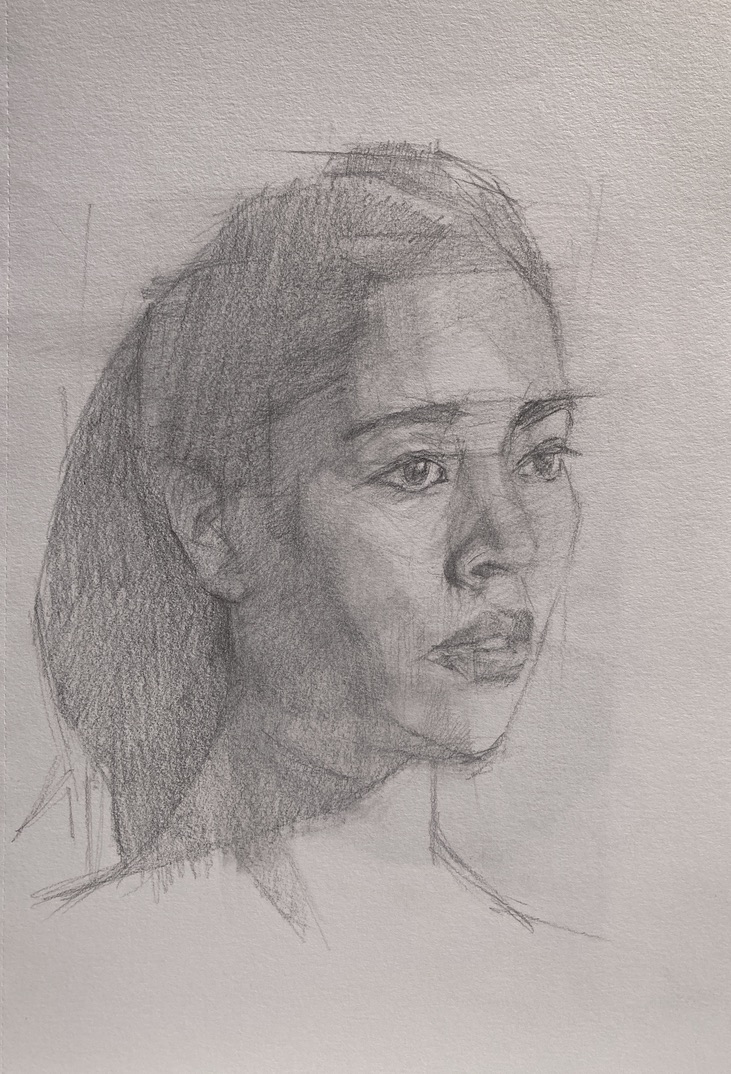The image depicts a realistic pencil sketch of a woman's face in a sketchbook. The paper is predominantly white with slight gray shadows and a textured surface, particularly noticeable at the top. The sketch primarily focuses on the woman's face and neck, with her form fading into white space below the neck. She is captured in a three-quarter profile, facing forward and to the right. Her hair is dark and pulled back into a ponytail that falls just below shoulder length. The drawing features her thick, dark lips, long eyelashes, and slightly sad expression. The intricate shading renders various dimensions to her nose, lips, eyebrows, chin, forehead, and cheeks, with darker shadows on the left side due to light coming from the right. There is no signature or text visible, and some rough sketch lines indicate the drawing might be unfinished. The shading scheme is detailed and complex, reflecting the artist's skillfulness. Her ear is visible against her dark hair, adding to the depth and realism of the sketch.